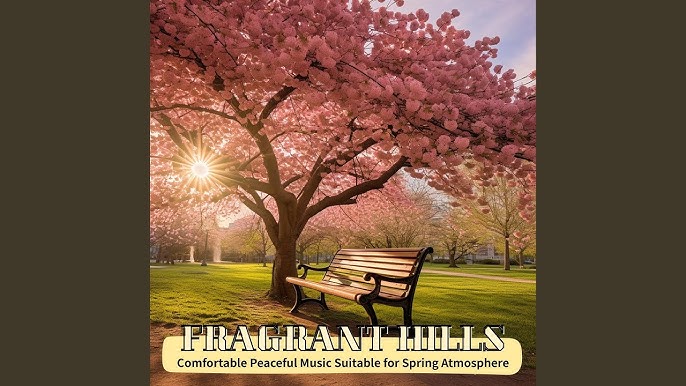The photograph, which appears to be the album cover for "Fragrant Hills," showcases a tranquil park scene suitable for the album's theme of comfortable, peaceful music for a spring atmosphere. At the foreground, there's a wooden park bench positioned next to a tree adorned with deep pink clusters of cherry blossoms, reminiscent of small puffs connected to the branches. This tree, along with several similar cherry blossom trees in the background, is bathed in sunlight, which beams gracefully through the branches, casting a warm glow over the well-trimmed, bright green grass. The serene setting is completed by additional trees lining a nearby sidewalk, all contributing to the inviting and peaceful ambiance of the photograph.